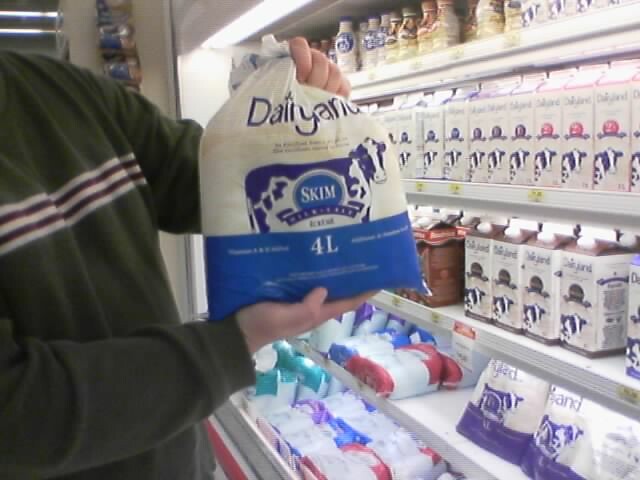In the dairy section of a grocery store, a man stands on the left side of the frame. His face is obscured, but his torso and arms, clad in a green sweater adorned with white and red stripes across the chest, are visible. He is holding up a Dairyland bag, which features an illustration of a blue cow and the label "skim." Though some text is not legible, the "4L" at the bottom suggests the bag contains four liters of a dairy product, likely milk. Below, a variety of similar bags in different colors are displayed, along with several cartons of milk neatly arranged on the shelves above.